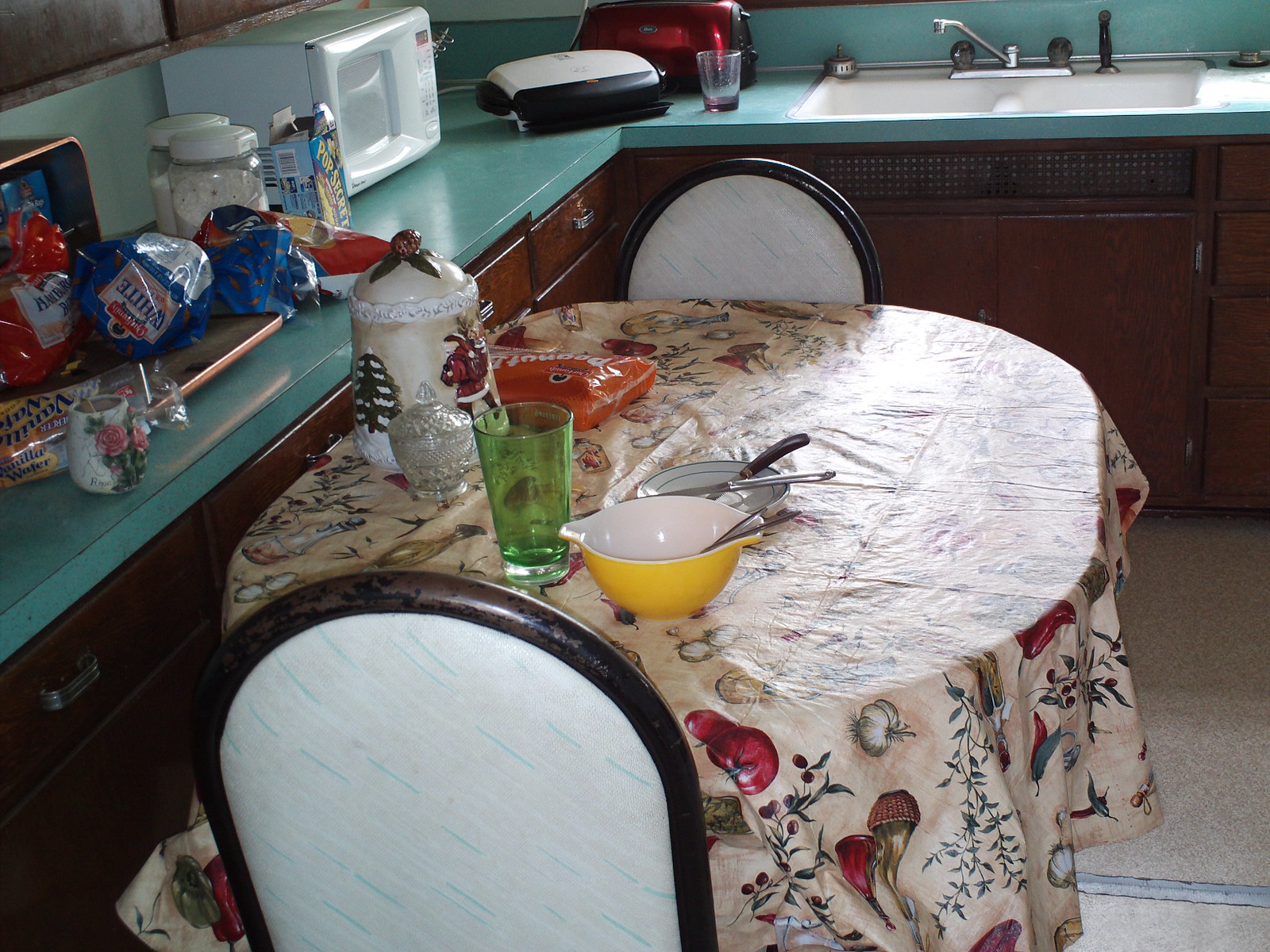The image captures a cozy yet cramped kitchen brimming with character and color. The countertops are a soft baby blue, contrasting with the timeworn brown cabinets that speak to their age. A large white sink anchors the workspace, accompanied by a white microwave and what appears to be a toaster. Various bags, likely containing bread, and canisters for storage clutter the countertops, adding to the sense of busyness.

In the limited space, a small kitchen table squeezes in, covered with a tablecloth adorned with vibrant plant, greenery, and bird motifs. The table is surrounded by white chairs edged with black, echoing the eclectic nature of the room. On the table, a green glass, a yellow bowl with a spoon, a small plate with a fork, and a canister matching the tablecloth’s design add to the colorful tableau. An orange bag and other small items also lay on the table, contributing to the overall crowded feel.

Despite its confined space and vintage appearance, the kitchen exudes a warm, almost retro-modern charm, accentuated by the striking blue cabinetry and the colorful assortment of everyday items.